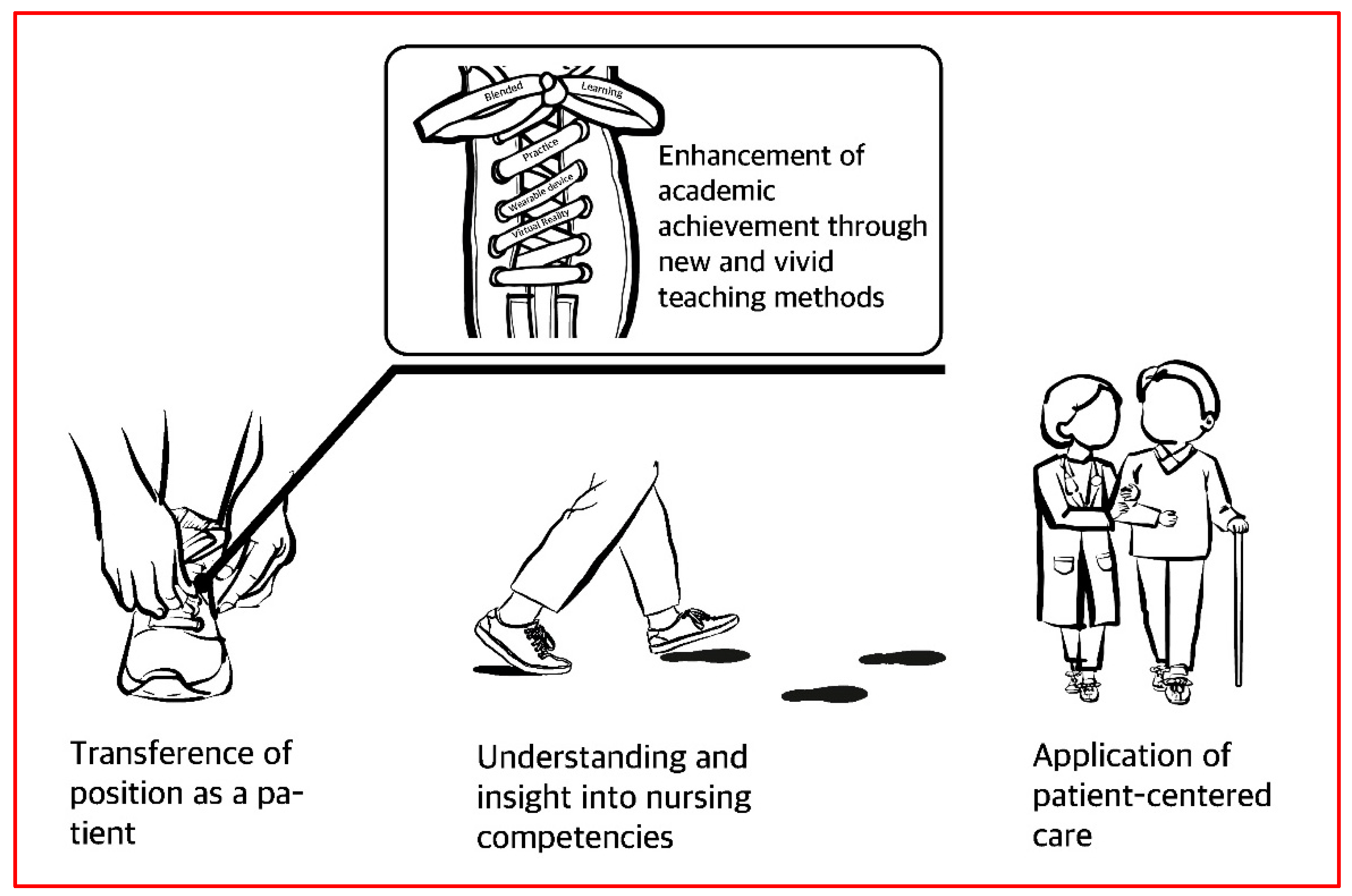This black and white image appears to be a detailed diagram, bordered in red, illustrating various aspects of nursing competencies and patient care. 

At the top center, there is a drawing of a shoe’s upper part, accompanied by the caption: "Enhancement of academic achievement through new and vivid teaching methods."

On the bottom left, the diagram depicts two hands tying a shoelace with the caption: "Transference of position as a patient."

In the center, the image showcases two legs walking with footprints leading ahead, underlined by the words: "Understanding and insight into nursing competencies."

At the bottom right, there is an illustration of two individuals walking. The person on the left, who appears to be a woman, is leading a person on the right, who seems to be a man using a cane. This section is labeled: "Application of patient-centered care."

The entire diagram is enclosed within a striking red border.